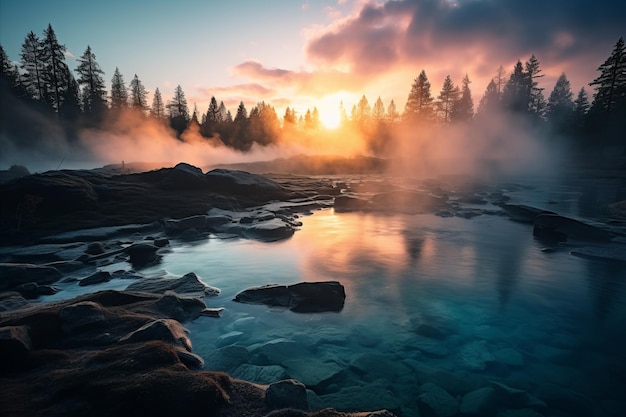The image depicts a serene sunset over a calm lake, bordered by a dense forest of tall pine trees. The sky, painted in shades of pink, yellow, and golden brown, captures the warm hues of the setting sun just above the horizon. To the left, the sky is remarkably clear. A thick layer of fog and mist drifts in front of the trees, adding an ethereal quality to the scene. The lake mirrors the sun, clouds, and surrounding trees in its still waters, enhancing the tranquil atmosphere. The shoreline is rocky, lacking any sandy beach, with various rocks and boulders scattered both in and around the water. The overall impression is one of natural beauty and calm, reminiscent of a digitally generated or AI-created landscape.